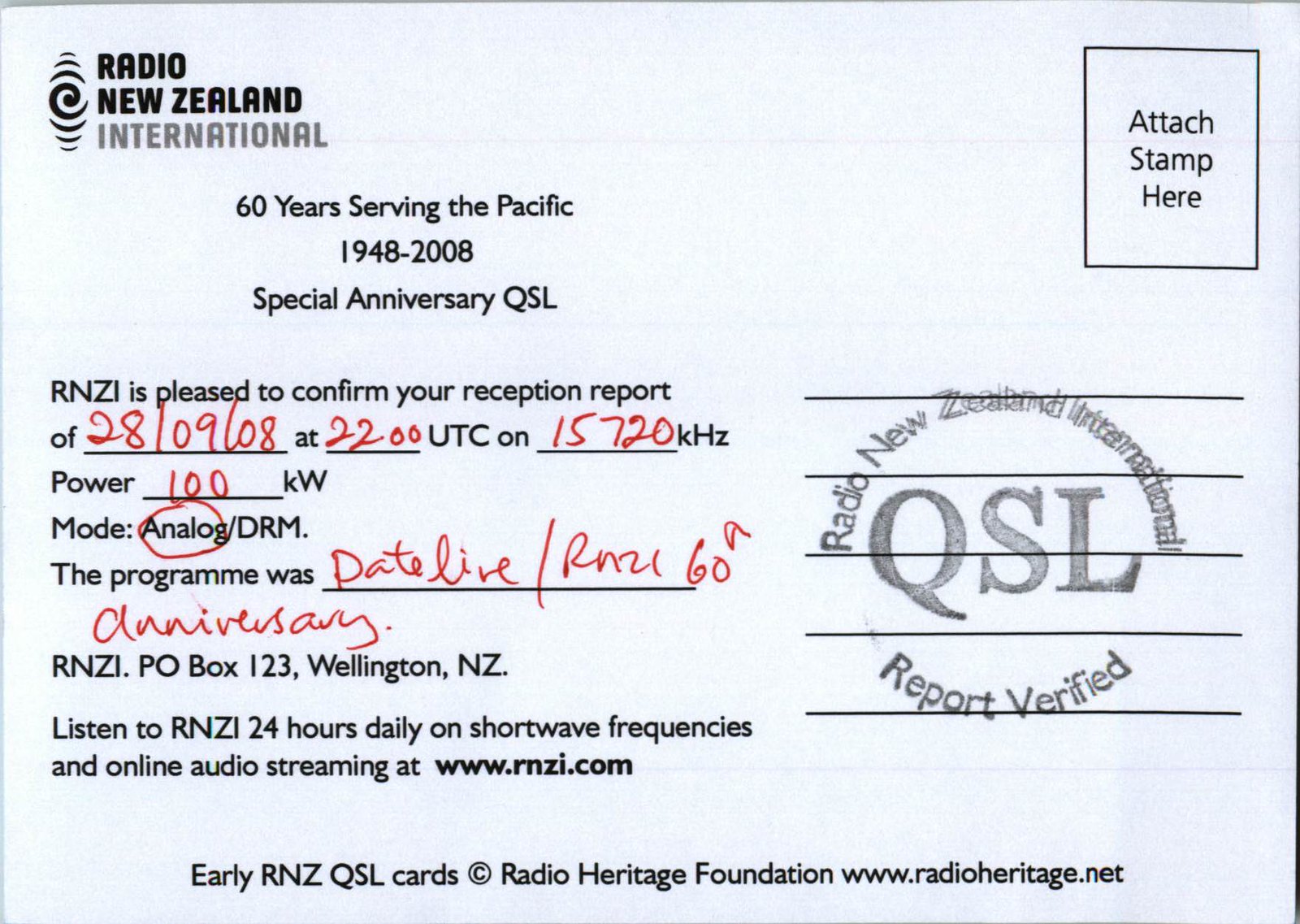The image depicts a special anniversary QSL postcard from Radio New Zealand International (RNZI), commemorating 60 years of service to the Pacific from 1948 to 2008. In the top left corner, the RNZI logo is prominently displayed, with "Radio New Zealand International" in black font, except for the word "International," which is in gray, adjacent to a swirly symbol. Below this, the postcard announces, "60 years serving the Pacific 1948-2008 special anniversary QSL."

On the top right corner, there is a black box labeled "Attach stamp here." Underneath the anniversary text, the postcard confirms a reception report with the handwritten details: "28/09/08 at 2200 UTC on 15720 KHz, Power: 100 KW, Mode: Analog/DRM," where "Analog" is circled in red. The program verified is "Dateline/RNZI 60th Anniversary."

Further text indicates, "RNZI is pleased to confirm your reception report," followed by the RNZI postal address: "RNZI, PO Box 123, Wellington NZ." Additional information invites listeners to tune into RNZI 24 hours daily on shortwave frequencies and online audio streaming at www.rnzi.com.

On the right side, the words "Radio New Zealand International" arc above the centrally placed term "QSL," and below that, "Report verified" arcs in a circular manner, resembling a stamp. At the bottom, it notes, "Early RNZI QSL cards" from the Radio Heritage Foundation at www.radioheritage.net. Some elements, including key reports and programs, are highlighted in red marker.